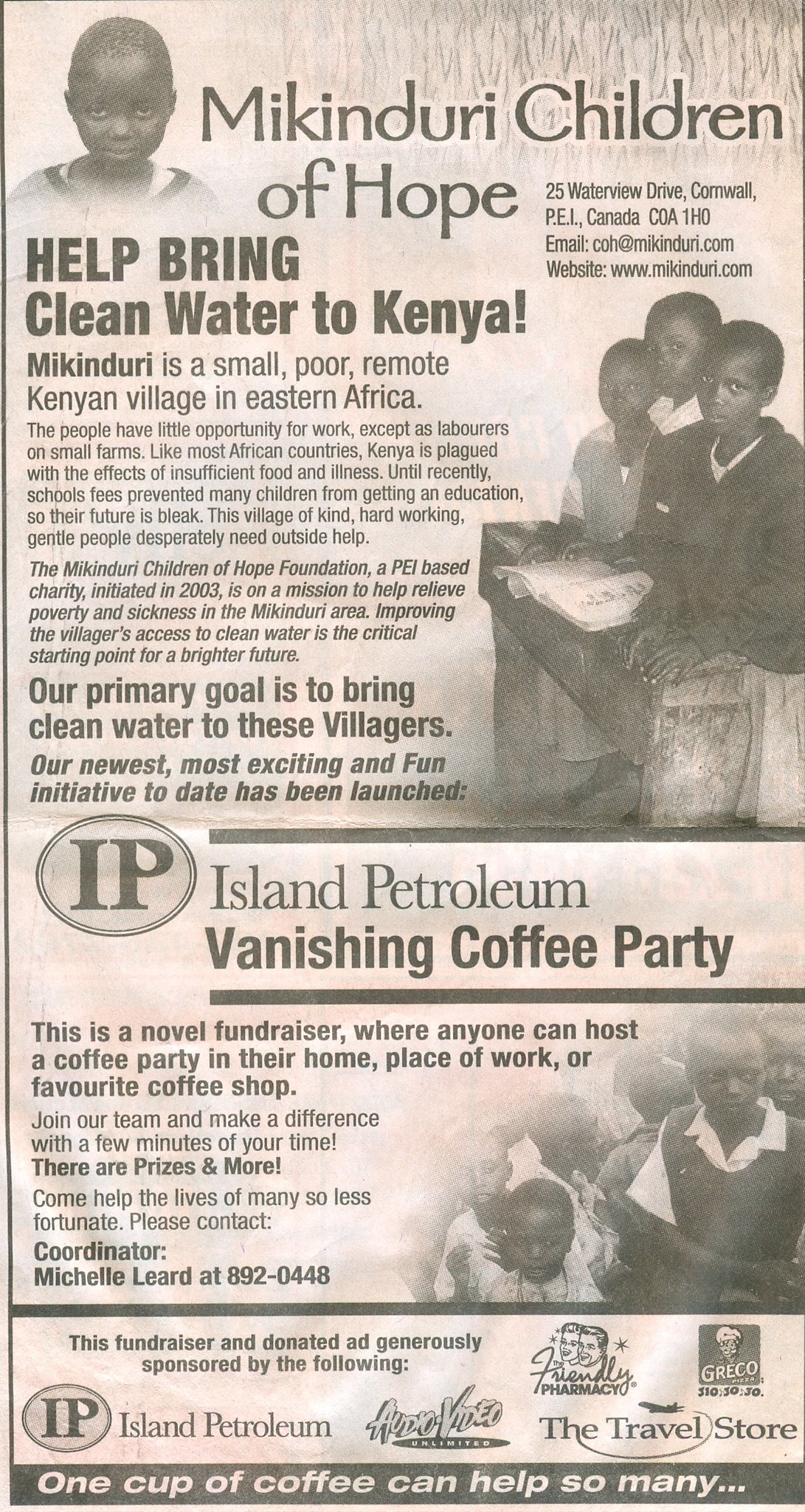This image depicts a black-and-white newspaper clipping or flyer with a slight sepia tone, featuring an appeal from the "McAndory Children of Hope" foundation. The clipping prominently highlights the foundation's mission to bring clean water to McAndory, a small, poor, remote village in Eastern Africa, plagued by insufficient food, illness, and limited educational opportunities. In its endeavors to alleviate poverty and sickness, McAndory Children of Hope, a PEI-based charity initiated in 2003, has organized a novel fundraiser called the "Vanishing Coffee Party." This initiative encourages individuals to host coffee parties in their homes, workplaces, or favorite coffee shops, aiming to gather support and resources for these villagers. The flyer includes images of impoverished Kenyan children and provides contact information: 25 Waterview Drive, Cornwall PEI, Canada COA 1H0, email coh@mcindory.com, and website www.mcandory.com. At the bottom, several sponsors like Island Petroleum, Audio Video Unlimited, Friendly Pharmacy, The Travel Store, and Greco Pizza are acknowledged, emphasizing that one cup of coffee can significantly help those less fortunate.